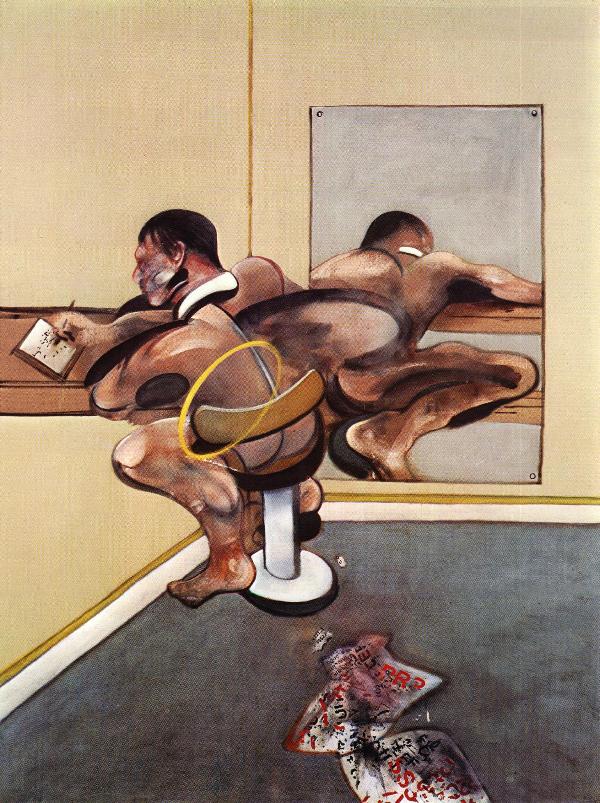The image is an abstract painting illustrating a man seated on a barstool-like chair, leaned over a brown counter, writing on a notepad. He has short hair and is unclothed, showcasing some muscular definition, with his bare back visible. The setting is a corner where two intersecting yellow walls meet. Behind him, on the back wall, is a mirror that reflects the scene, though the reflection is somewhat blurred. The man is positioned in the left corner of the room. The floor is carpeted in gray, with crumpled pieces of paper with black and red writing scattered towards the front. The room features a palette of grayish-green, red, black, white, brown, tan, beige, and light yellow colors, creating a cohesive and detailed portrayal of the man absorbed in his writing task.